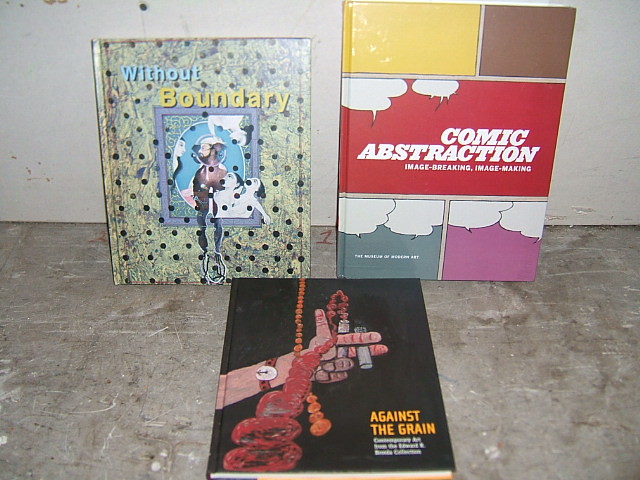Three books are arranged on a worn, gray concrete floor against a beat-up white wall. Two books, titled "Without Boundary" and "Comic Abstraction: Image Breaking, Image Making," are leaning against the wall, while the third book, "Against the Grain," lies flat in the foreground. 

The "Without Boundary" book features a modern art cover with a green backdrop resembling foliage, adorned with black polka dots. Within the frame at the center of the cover, there are four women observing a creature with a man-like face and bird-like talons.

The "Comic Abstraction: Image Breaking, Image Making" book has a cover divided into colorful blocks. These include a yellow triangle, a brown square, a red triangle, a blue square, and a pink square, each containing comic word bubbles. The title is prominently printed in white block letters.

"Against the Grain," the book lying flat, has a black cover depicting a hand from the elbow up, wrist adorned with a watch, holding two cigarettes. Red smoke emanates from the cigarettes, providing a striking visual effect. The title is presented in yellow block letters in the lower right-hand corner. 

The arrangement of the books on the industrial floor against the weathered wall creates an interesting visual juxtaposition, emphasizing the eclectic nature of the collection.